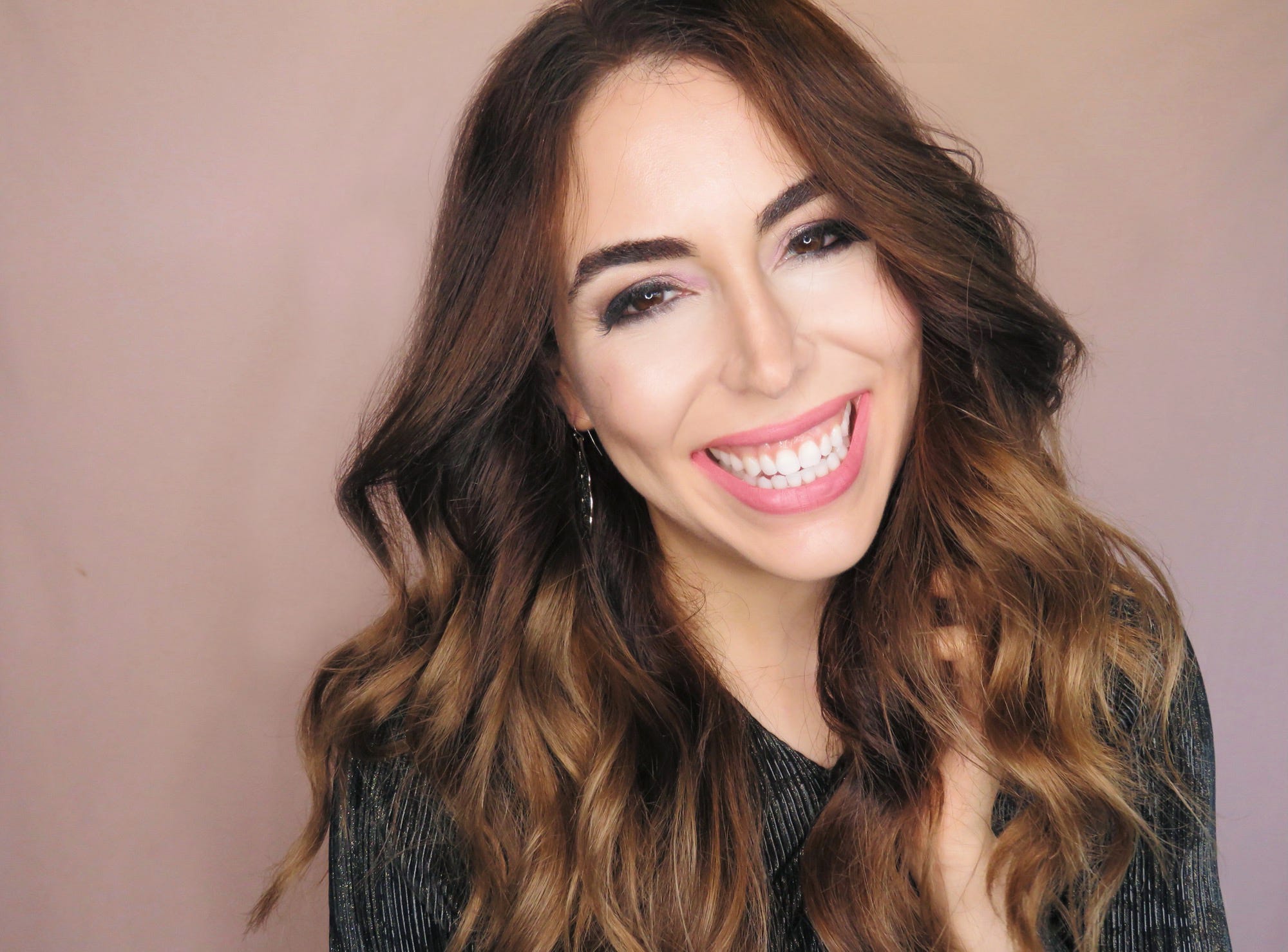This captivating headshot features a cheerful young woman with a radiant smile, revealing her bright white teeth. She has dark brown eyes framed by equally dark eyebrows, complementing her fair white complexion. Her long, wavy brown hair cascades below her shoulders and shows hints of lighter ends. A subtle curl adds volume and texture to her hairstyle. She is wearing a black and white striped blouse, with the vertical stripes being very subtle and occasionally highlighted by streaks of shiny silver. Her makeup is well-applied, including pink lipstick that accentuates her smile. She is also wearing earrings, adding a touch of elegance to her appearance. Her head is slightly tilted, and one of her hands is grasping at her hair, adding a candid feel to the image. The background is a solid gradient of pinkish-mauve, with a centralized light illuminating her face. The reflection of this ring light is visible in her eyes, suggesting a professional setup that enhances the clarity and overall quality of the photograph. The vibe of the image suggests she might be preparing for a special occasion or a professional photo shoot.